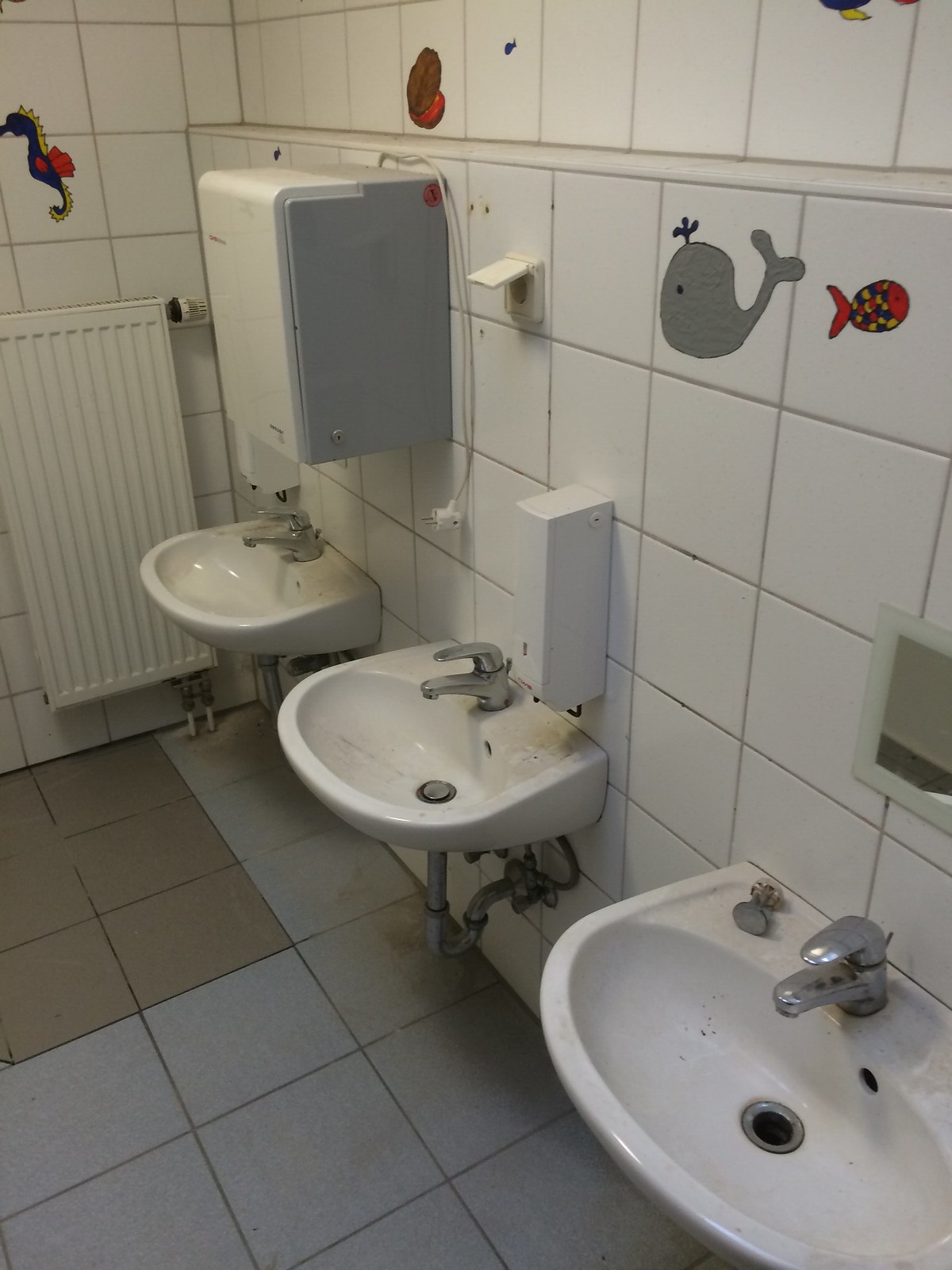This photograph captures a children's public bathroom, likely located in an elementary school, as indicated by the low-set sinks tailored for kids. The bathroom features a light gray and brown-tiled floor and walls adorned with white tiles. A variety of vibrant sea life decals brightens up the space, including a gray whale, a red fish, a brown clam with a red interior, and a blue seahorse. These playful decorations contribute to the child-friendly ambiance.

There are three white sinks equipped with silver nozzles, suggesting frequent use due to their visible wear. The central sink has a push-button tap mechanism for water. Above each sink, there are soap dispensers, with the one above the middle sink being explicitly mentioned. To the left of these sinks, there's a white radiator providing heating. Additionally, a hand towel dispenser is fixed above the sink on the left. The detailed elements and the careful arrangements underscore the functional yet engaging environment designed for children's use.